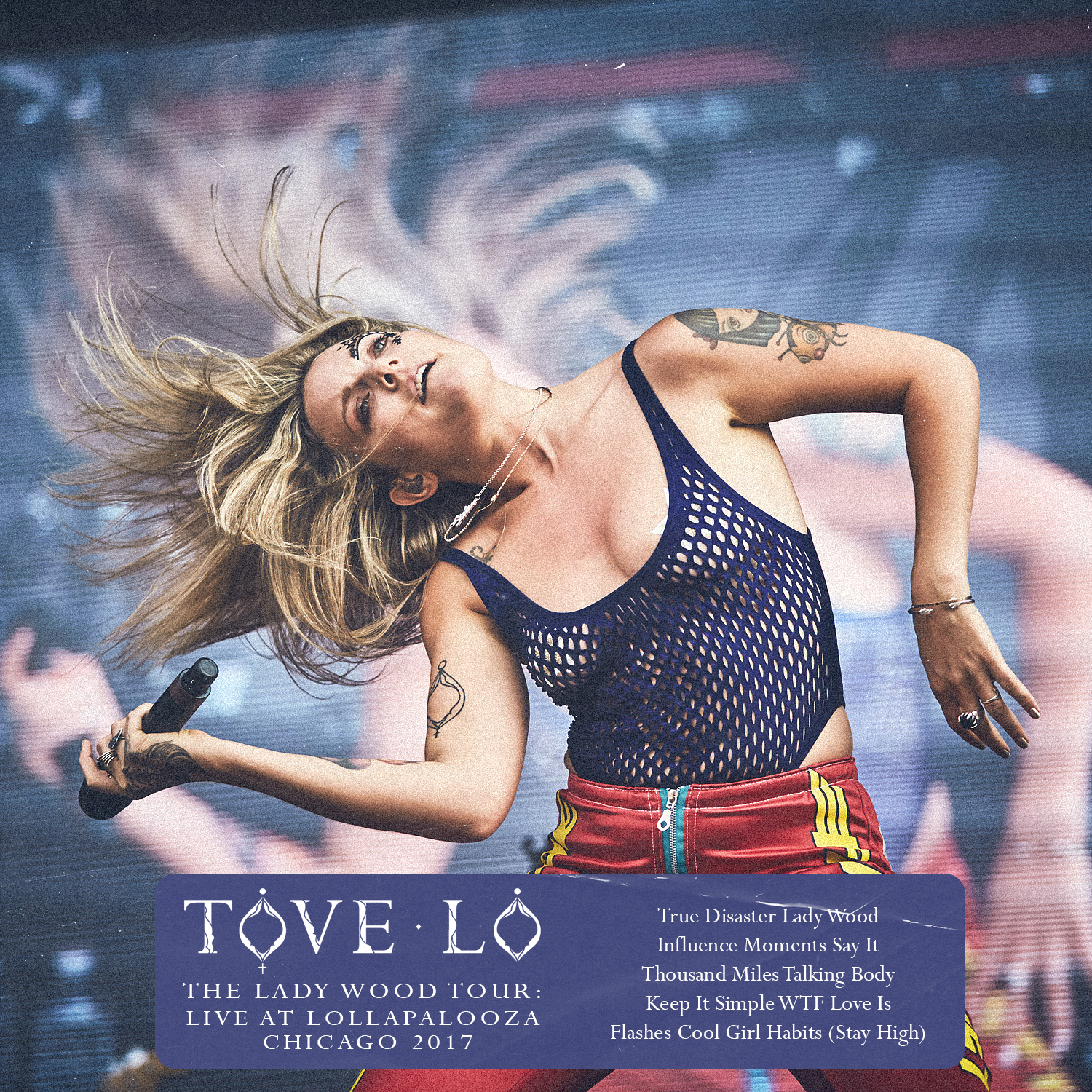This image features a dynamic and energetic performance advertisement from the Lady Wood Tour, headlined by Tove Lo at Lollapalooza in Chicago, 2017. The central figure is a blonde Caucasian woman, captured in mid-action with her hair flying to the side, which conveys a sense of movement as she rocks out on stage. She is holding a black microphone in her right hand and wears a distinctive ensemble: a see-through navy blue fishnet tank top paired with red pants that feature yellow stripes down the sides and a blue zipper. The woman is adorned with several tattoos including a cartoon girl on her left shoulder, and others on her right collarbone, bicep, and forearm. Additionally, she has tattoos or black face paint on her left eyebrow and beneath her left eye.

Her accessories are notable, including a silver necklace, a silver bracelet, and silver rings on her left hand. Behind her, a large screen displays her live performance and dance moves. A blue square text box at the bottom of the image reads, "Tove Lo, The Lady Wood Tour Live at Lollapalooza Chicago 2017," followed by a list of song titles: "True Disaster," "Lady Wood," "Influence," "Moments," "Say It," "Thousand Miles," "Talking Body," "Keep It Simple," "WTF Love Is," "Imaginary Friend," "Cool Girl," "Habits," and "Stay High." This detailed scene captures the exuberance and visual aesthetic of Tove Lo's live performance, promising an unforgettable concert experience.